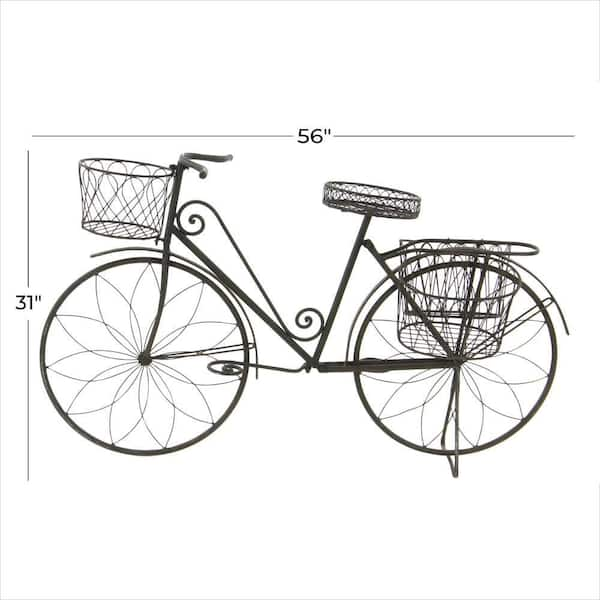The image depicts a black and white diagram of an antique-style bicycle repurposed as a decorative garden feature, likely made entirely of wrought iron. The bicycle measures 56 inches in length and 31 inches in height. The wheels are adorned with floral-patterned metal spokes instead of typical spokes, and the bicycle is held upright by a metal stand affixed to the rear wheel. This decorative piece features several swirled metal designs integrated into the frame. It has multiple planters: a metal basket on the handlebars, a metallic seat that doubles as a planter, and two metal baskets on either side of the rear wheel. Notably, the bicycle lacks functional pedals, emphasizing its sculptural and ornamental purpose. The background is primarily flat white on the left-hand side, highlighting the intricate design of the bicycle.